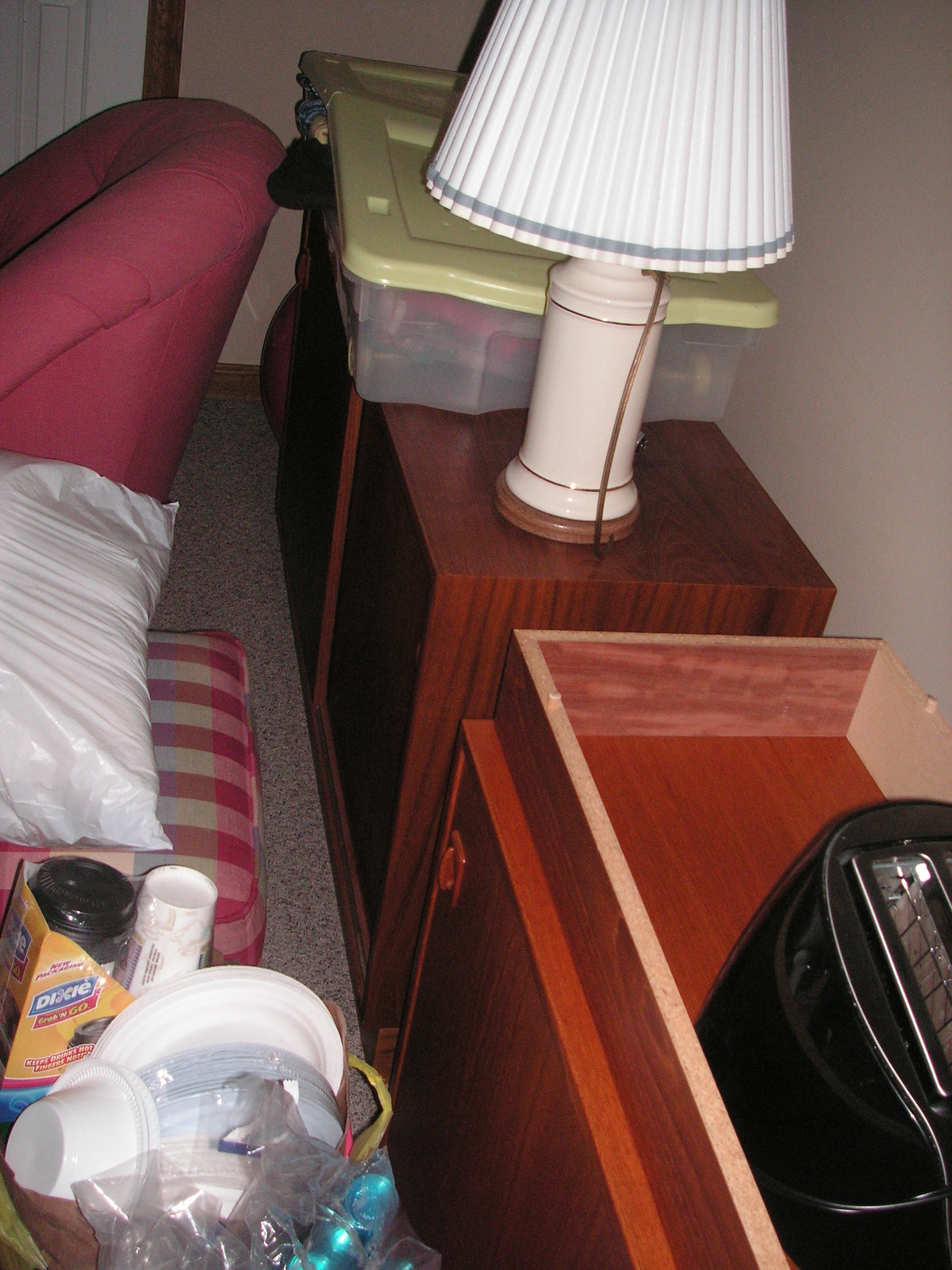The image depicts an overhead view of a room featuring a variety of items and furniture. Dominating the wall is a dark wooden cabinet devoid of doors, exposing its contents. The walls are a soft cream color, providing a warm contrast to the dark wood. Perched on the cabinet is an elegant white lamp adorned with gold lines at the top and bottom. The lamp’s shade is also white, accented with a grayish line at the bottom.

Adjacent to this cabinet is a smaller one, and next to it sits a sleek, thin plastic box with a light green cover. A toaster is visible in the corner, hinting at the room's likely function as a kitchen or multipurpose space.

In the lower portion of the image, part of a red chair is visible, accompanied by a checkered ottoman in red and white. On top of the ottoman, there's a white plastic bag, and in front of it lies a small pile of disorganized items, including a plate, various plastic pieces, bottles, and an unopened package containing a bottle.